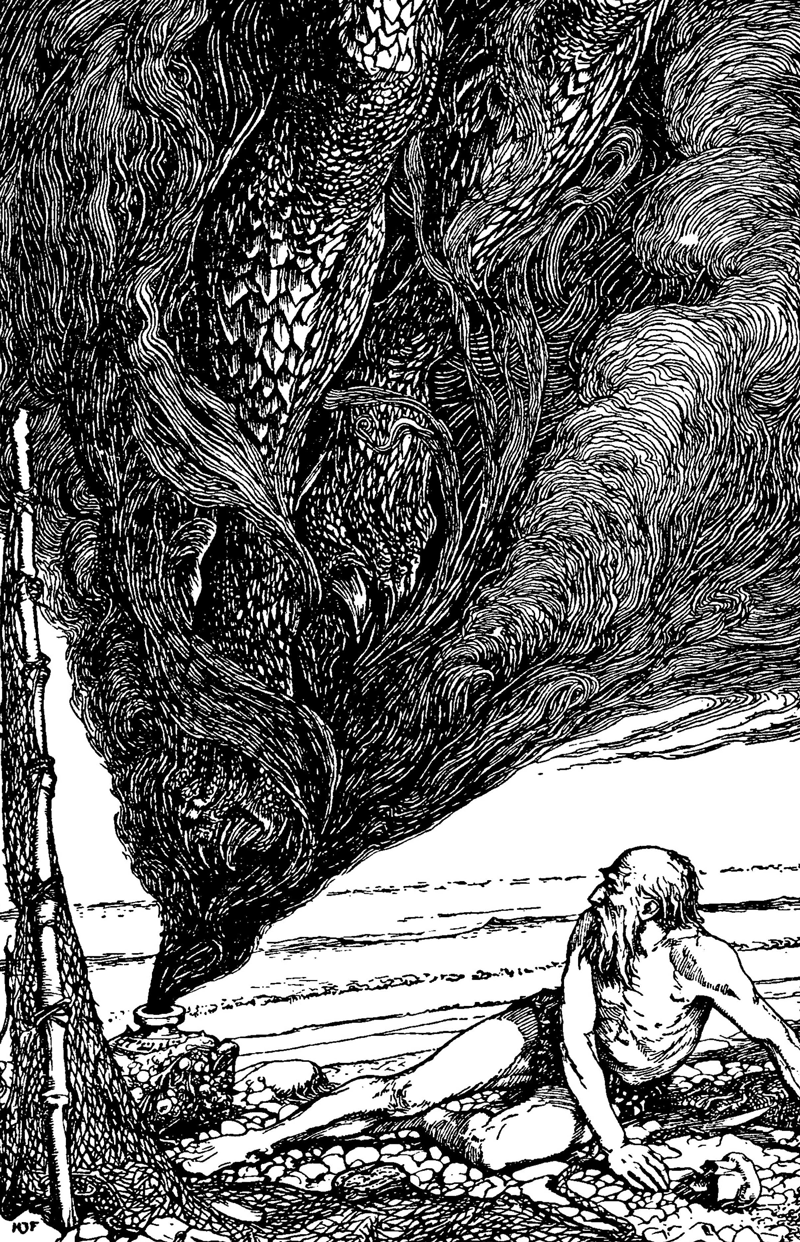This rectangular black-and-white drawing, approximately six inches high and three inches wide, depicts a distressed, shirtless man with long, scraggly hair and a beard, sitting on a rocky shore. His gaunt frame reveals prominent ribs and defined, albeit skinny, muscles, suggesting malnourishment. The man appears aghast, staring at an open pot or bottle beside him, from which a swirling miasma of smoke and patterned lines emerges. Within the smoky tendrils, partially obscured scaly legs and feet hint at a genie or mystical creature. Behind the man, ocean waves crash against the rocky beach. To the left of the scene, the base of a tree trunk holds a long fishing pole, and a net is placed nearby. The detailed, intricate lines and shading of the drawing enhance the sense of desolation and surprise captured in the scene.